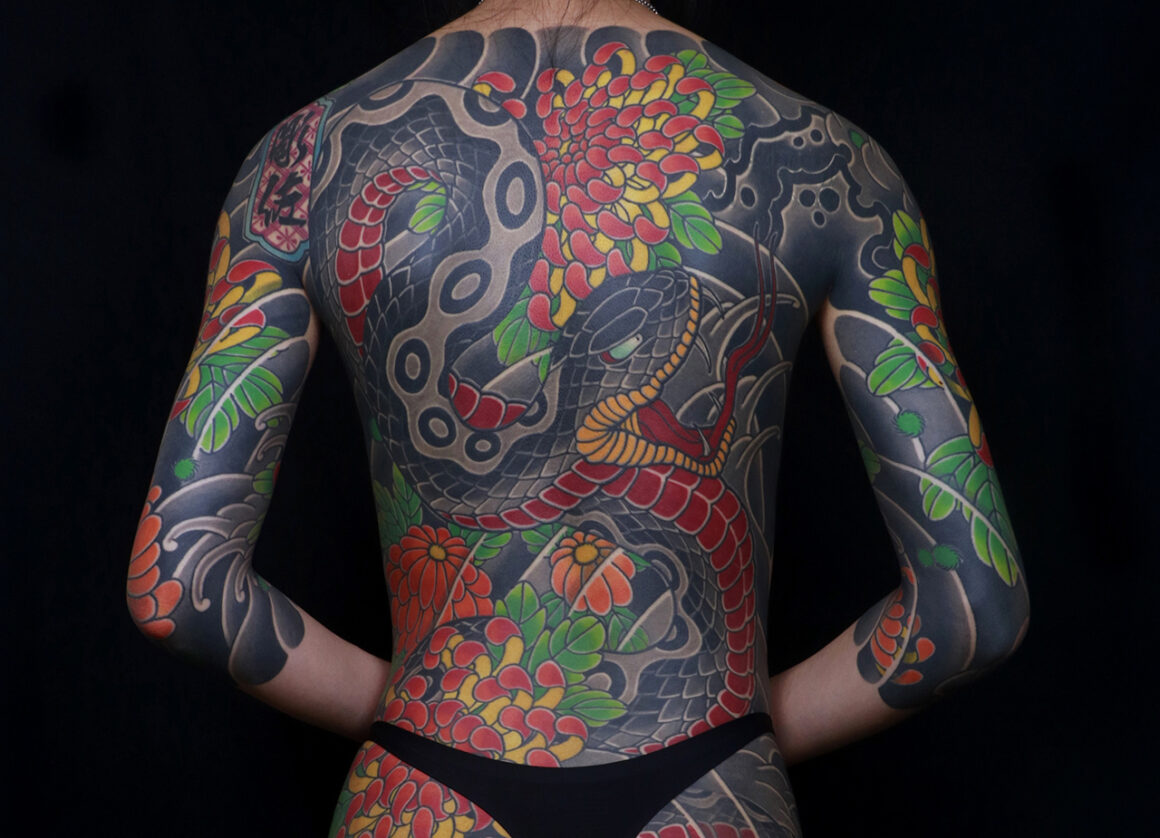The image features the back of a person with an extensive and intricate full-body tattoo in a traditional Japanese style, captured against a black background, suggesting a professional photo. The tattoo covers almost every inch of the person's back, reaching from the legs up to the collarbone, leaving only the neck and wrists untouched. The centerpiece of the tattoo is a highly detailed and articulated snake, coiled in an elaborate design. The snake has a black body with grayish round shapes, a belly made up of red scales, a yellow-orange mouth, green eyes, and a long, forked red tongue. Surrounding the snake are vibrant red and yellow flowers, interwoven with dark black clouds, green leaves, and other intricate patterns, creating a mosaic-like effect. Additional details include chain-like patterns along the snake's back, which contribute to the overall elaborate and masterful design. A glimpse of white skin and brown hair can be seen at the neckline, accentuating the comprehensive coverage of the tattoo.